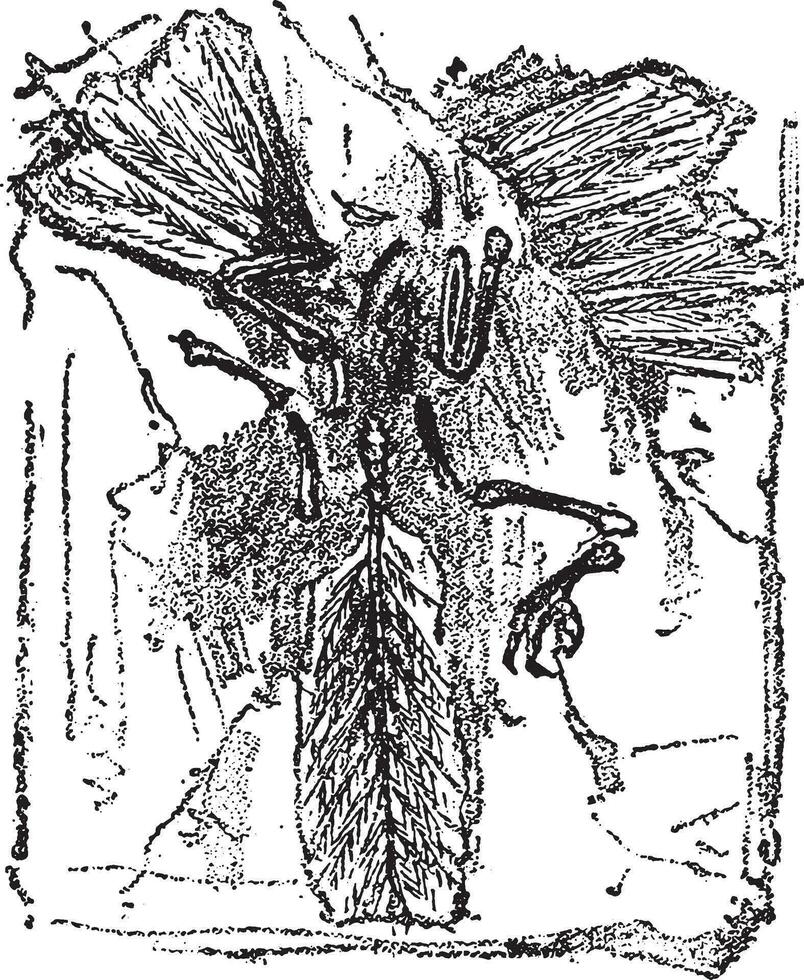The image is a complex black and white drawing, predominantly in a scribbly, pointillism, or charcoal style. The central subject appears to be a rough sketch of a decayed or mangled mythical creature, possibly a bird or insect. The middle is chaotic, featuring a discernible spine or bone structure flanked by skeletal arms or legs, one of which culminates in a claw seemingly clutching a leaf on the right. At the top, there are arcs or shapes reminiscent of peacock feathers or wings, suggesting a tattered and confusing outline, further adding to its enigmatic nature. The image has a patchy black border, and the lower portion possibly depicts a large leaf or insect-like body. Some interpret a bird's beak and eyeball within the jumbled forms, reinforcing the figure's monstrous and fossil-like appearance. Overall, it is an antiquated, ambiguous depiction of a creature that invokes interpretations ranging from a bird to a decayed insect, wrapped in abstract, erratic strokes and dense texturing.